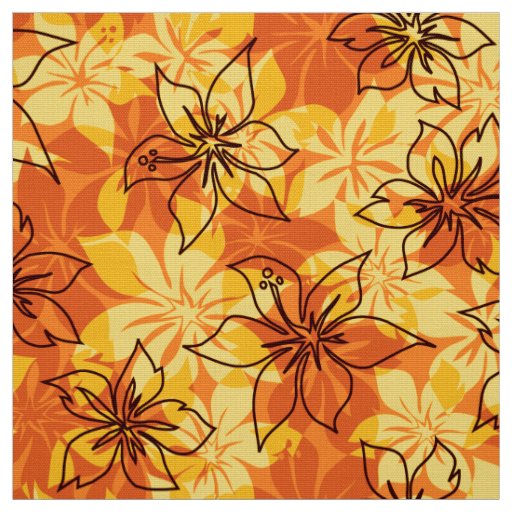This image features a vibrant, tropical floral pattern that could be used on various beach-related items such as bathing suits, beach towels, surfboards, or even wallpaper and fabric. The design is rich with overlapping flower shapes in different shades of yellow, golden-yellow, burnt orange, and off-white, set against a reddish-orange background with hints of peach. The most prominent elements are black-outlined hibiscus or similar-style flowers, complete with upward-sticking stamens, juxtaposed against background flowers that resemble lilies or hibiscus. The layering of colored and outlined flowers creates a sense of depth and complexity, giving the pattern a dynamic and uplifting feel. This detailed, multi-layered design evokes a sense of tropical vibrancy and artistic flair.